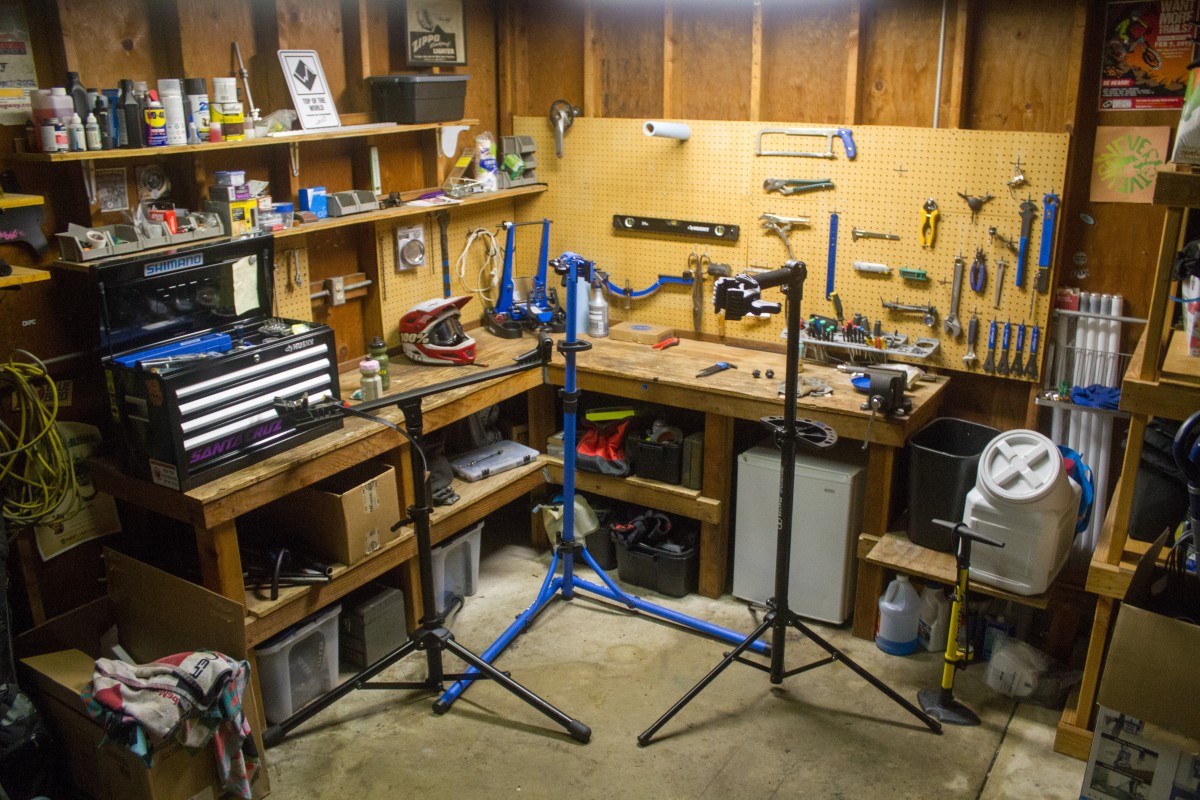This color photograph captures the corner of a cluttered garage workshop, showcasing a meticulously organized yet heavily utilized workspace. Prominently featured is a wooden L-shaped workbench with a rough, handmade appearance, complete with a middle shelf and plastic storage containers beneath it. Atop the bench rests a black toolbox with multiple drawers, alongside a red and white motorcycle helmet.

The back wall is dominated by a pegboard densely populated with various tools, including a handsaw, level, pliers, and wrenches of different sizes. Attached to one end of the workbench is a vise, while the other end houses a small mini white refrigerator. Numerous shelves, under which bins and totes are slid, hold garage staples like cans of WD-40, paint thinner, and spray paint. The room is also equipped with freestanding jacks and a shop light, adding to the impression of a well-stocked and versatile workspace.

An extension cord hangs on the left wall, and a container full of hand tools such as screwdrivers is positioned on the work surface. The floor is scattered with stands that might serve for photography or lighting purposes, contributing to the overall impression of a multifunctional space dedicated to various DIY projects and maintenance tasks. The entire scene is a vivid representation of a busy, tool-filled garage.